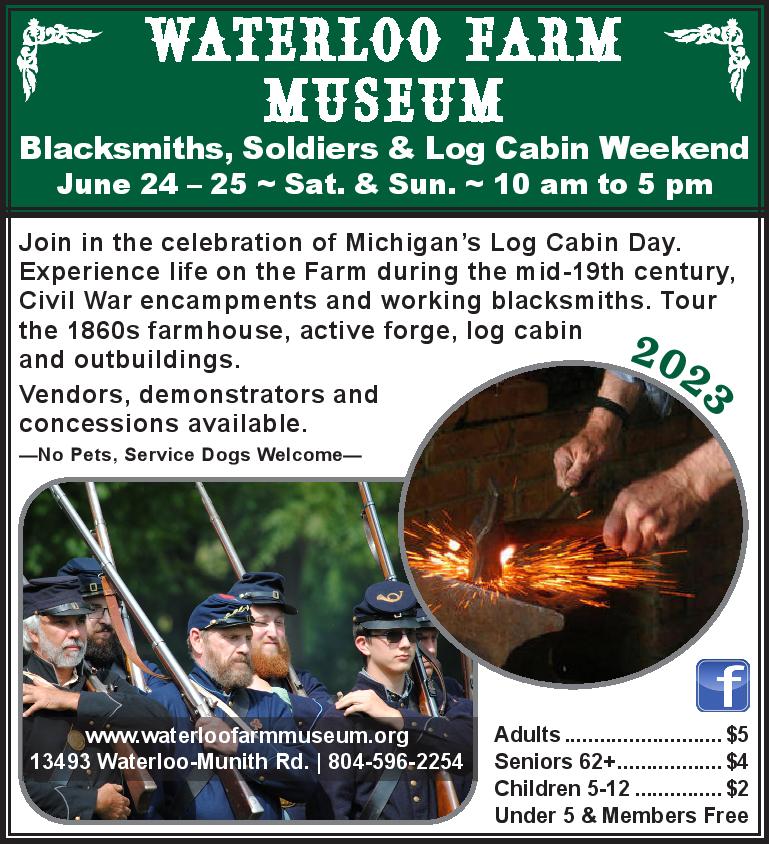The advertisement for the Waterloo Farm Museum event is visually captivating, featuring a combination of photography and graphic design. The poster is in a portrait orientation, divided into two main sections. The top section has a green background with white antique text that announces "Waterloo Farm Museum" framed by elegant flourishes on either side. Beneath this, still in white text, it elaborates the event's theme: "Blacksmiths, Soldiers, and Log Cabin Weekend," followed by the dates and times—June 24-25, Saturday and Sunday, 10am-5pm.

Separated by a thin black horizontal line, the lower section is set against a white background with detailed black text. It invites visitors to join in celebrating Michigan's Log Cabin Day and promises an immersive experience of mid-19th century farm life, including Civil War encampments and active blacksmith demonstrations. It lists several attractions such as the 1860s farmhouse, an active forge, outbuildings, and a log cabin, augmented by the presence of vendors, demonstrators, and concessions. It also notes that pets are not allowed, except for service dogs.

On the right side of this section is a circular photograph capturing a blacksmith in action, sparks flying as he hammers glowing metal on a rusty anvil, with red bricks visible in the background. Above this image, the year "2023" appears in green text. On the bottom left, there is a rectangular photograph of Civil War reenactors in blue uniforms and hats, featuring participants of varying ages, some with beards, one child notably wearing sunglasses. 

The poster also includes the museum's URL (www.waterloofarmmuseum.org), the address (13493 Waterloo Munith Road), and ticket prices—adults $5, seniors (62 and over) $4, children (5-12) $2, with free entry for children under 5 and members. Lastly, a blue and white Facebook logo is placed above the ticket information, indicating social media presence.